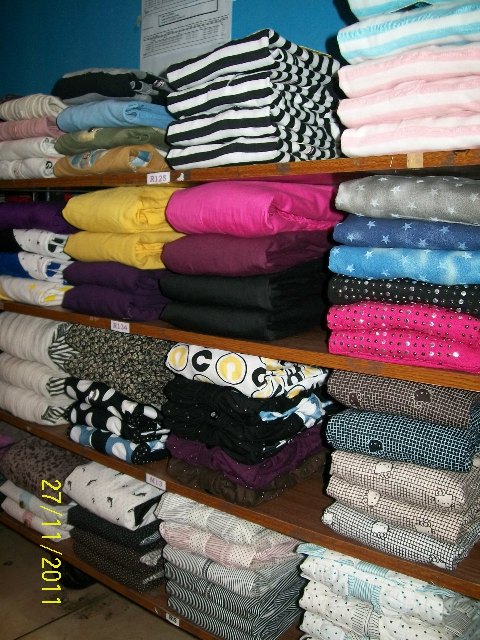In an indoor color photograph taken on 27-11-2011, we see a meticulously organized storage area, possibly within a fabric store. The main focus is on four wooden shelves, each laden with neatly folded piles of fabrics and shirts, showcasing a vibrant array of patterns and colors. There are solid color fabrics, as well as those with prints, herringbone patterns, stripes, plaids, and polka dots. Each pile typically consists of four items, suggesting a consistent arrangement. Notably, the shelves have numbers and tags for identifying different sections of the fabrics. The background wall, painted a bluish-green, features a taped instruction sheet that adds a functional touch to the space. The items look brand new, with some shirts in hues of yellow, pink, brown, and black, all folded precisely to maintain order. The image also includes a yellow overlay displaying the date "27/11/2011" in the lower left corner. The angle of the photograph, taken from the right, adds depth to the scene as the shelves angle slightly back to the left.